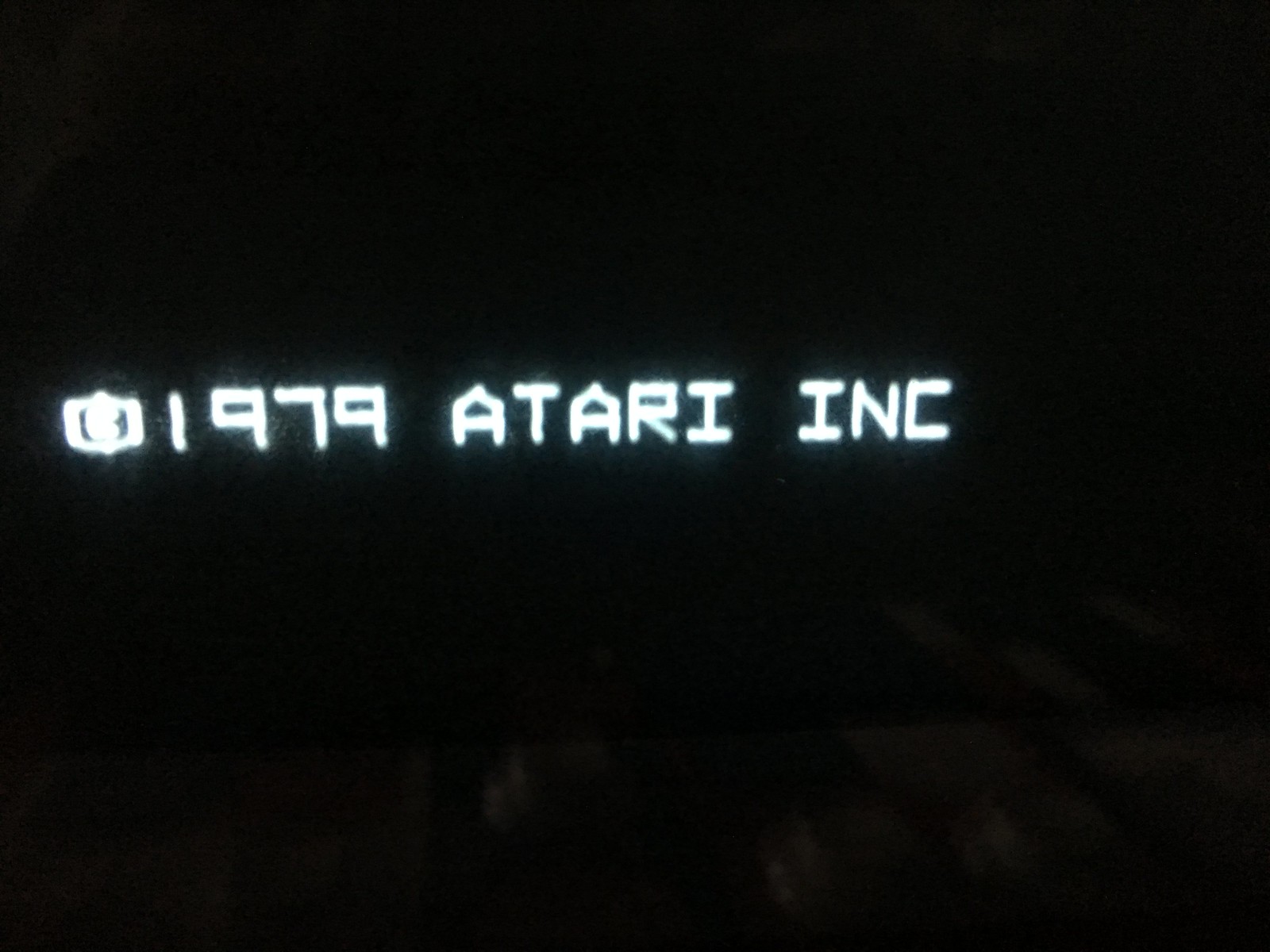This image features a black and white composition with a predominantly black background, punctuated by small, subtle smudges near the bottom, possibly in a brownish hue—suggesting it might be a colored image viewed in high contrast. At the center left, there is a notable white rectangular logo displaying a prominent 'C,' possibly indicating a copyright symbol. Below this logo, the text "1979 ATARI IMC" is rendered in a white, computer-esque font, evoking the aesthetic of early personal computer screens. The minimalistic and monochromatic design, along with the Atari reference, positions this image squarely within the technological landscape of the late 1970s or early 1980s, reminiscent of the simple graphics and text-based interfaces preceding the advent of modern, colorized operating systems.